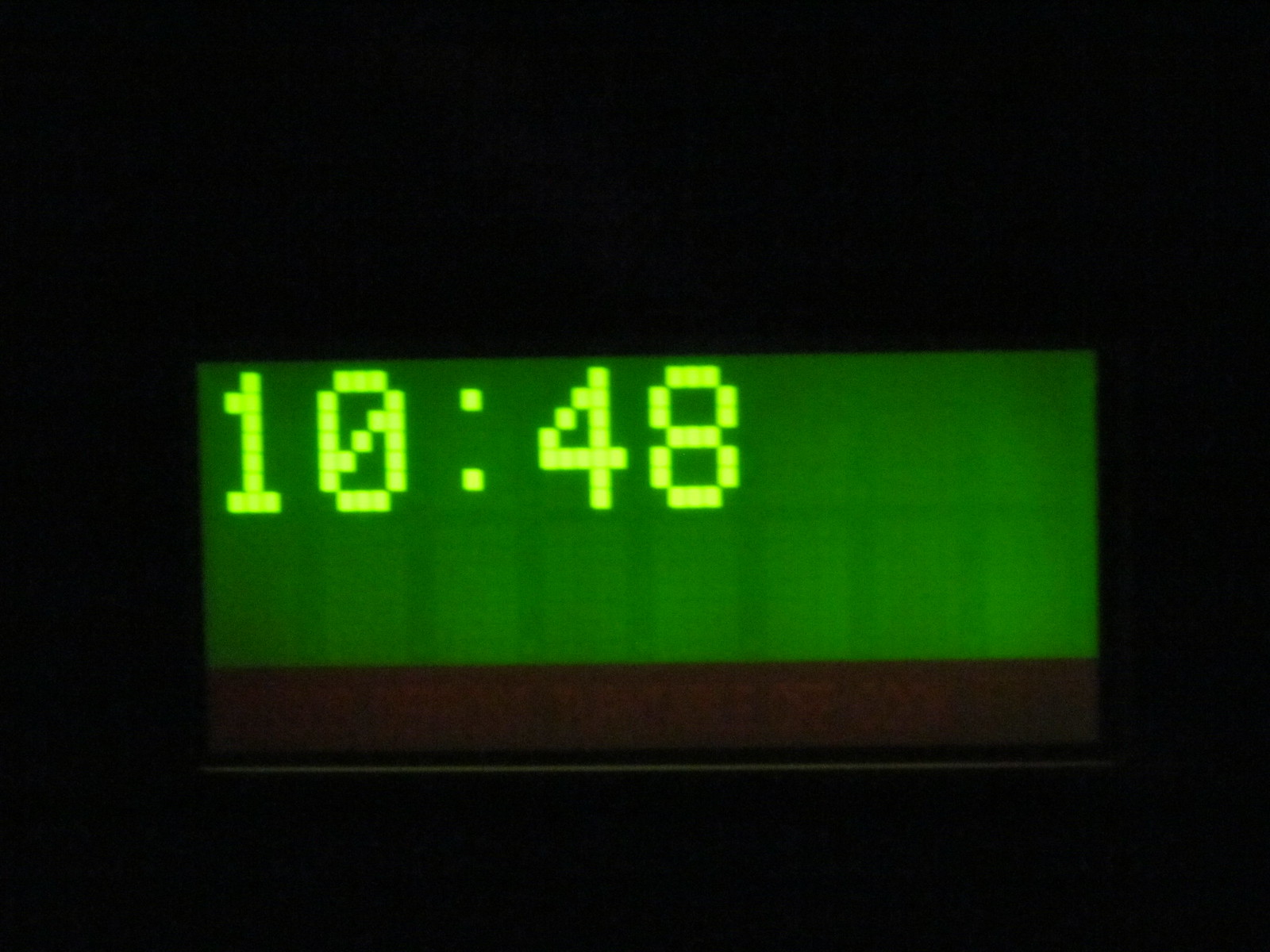This image features a striking digital clock set against a pure black background, highlighting its distinct form. The clock itself has a dark brown, nearly black, frame that seamlessly blends into the dim backdrop. The screen is a deep green hue, providing a subtle contrast to the darker surroundings. Displayed prominently in the center of the screen are large, luminous light green digits that read "10:48", making the time immediately readable even from a distance. The numerals are impressively sized, standing over an inch tall, which adds to their clarity and visibility. The harmonious color combination of light green digits on a dark green screen, bordered by the almost black edges of the clock, creates a visually captivating and easily legible display.